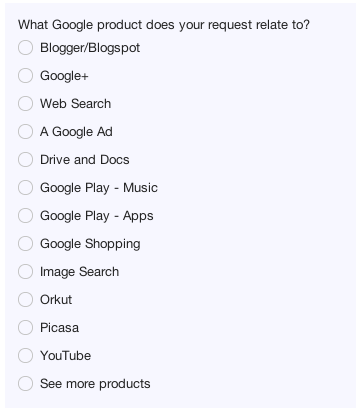The image depicts a light blue background with a visually structured questionnaire. The top part of the image features a question in light black text: "What Google product does your request relate to?" Below the question, there is a vertical list of options, each accompanied by an empty circle to the left. The listed options are:

1. Blogger/Blogspot
2. Google+
3. Web search
4. Google Ads
5. Drive and Docs
6. Google Play Music
7. Google Play Apps
8. Google Shopping
9. Image search
10. Orkut
11. Picasa
12. YouTube
13. See more products

None of the circles next to the options have been filled in, indicating that the questionnaire has yet to be completed. There is no additional text or context provided about the origin of the page, making it a straightforward snapshot of the questionnaire.